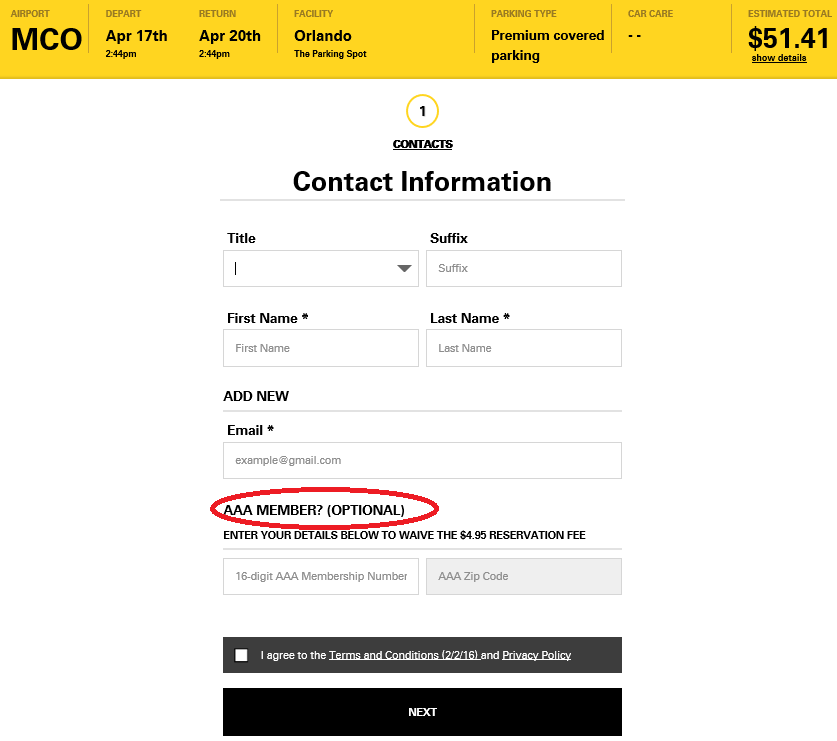Here is a detailed and cleaned-up caption for the image described:

---

This image appears to be a screenshot of a travel-related website, likely Hertz. At the top, a gold-colored horizontal bar spans the width of the screen, displaying the airport code "MCO" alongside the departure date and time of April 17th at 2:44 PM and a return date and time of April 20th at 2:44 PM. The facility is listed as Orlando, specifically 'The Parking Spot,' with the parking type designated as premium covered parking and no additional car care services. The estimated total cost is shown as $51.41. There is an option to click a button to "Show Details."

Below this section, labeled as "Number 1 - Contacts," fields for entering contact information are present. Users are prompted to provide their title and suffix, as well as first and last names, which are required fields. There is an "Add New" button followed by a required email field pre-filled with placeholder text "example@gmail.com."

Further down, there is a highlighted section marked by a red circle, which asks, "Are you an AAA member?" This is optional but indicates that entering membership details can waive a $4.95 reservation fee. Fields are provided to enter the membership number and zip code, and users must check a box to agree to the terms. Below this, there is a "Next" button to proceed.

---